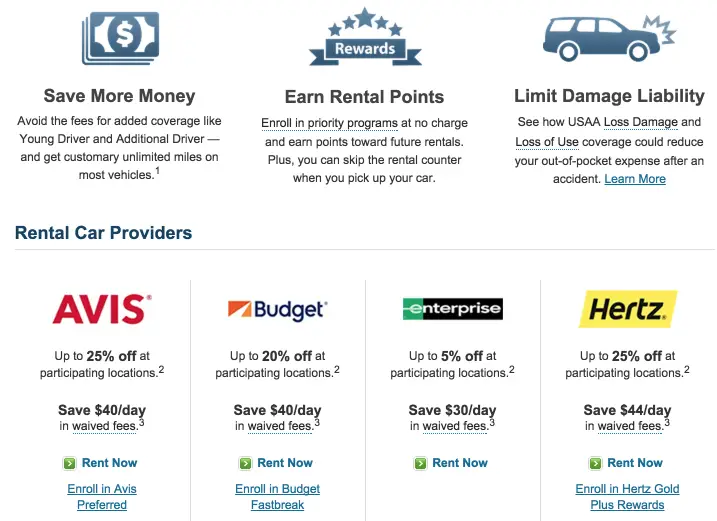A prominent advertisement by USAA highlights rental car services. The main focus is on a centrally placed vehicle image, with a detailed list of rental car providers below it. The advertisement banner is divided into three sections with bold headings: "Save More Money," "Earn Rental Points," and "Limit Damage Liability." Notably, under "Limit Damage Liability," it mentions USAA's Loss Damage Coverage.

Further down, the rental car providers listed include Avis, Budget, Enterprise, and Hertz. Each provider shows potential daily savings and available discounts for USAA members. There is also a "Rent Now" call to action button, accompanied by an option to enroll in a rewards program.

Interestingly, different icons above the "Save More Money," "Earn Rental Points," and "Limit Damage Liability" headings are visually muted in shades of blue, gray, and white without any vibrant colors. This subtle design choice sets a tone that is both professional and understated. It's also worth noting that among the providers, Enterprise lacks a specific loyalty program compared to competitors like Hertz, which features a "Gold Plus Rewards" program.